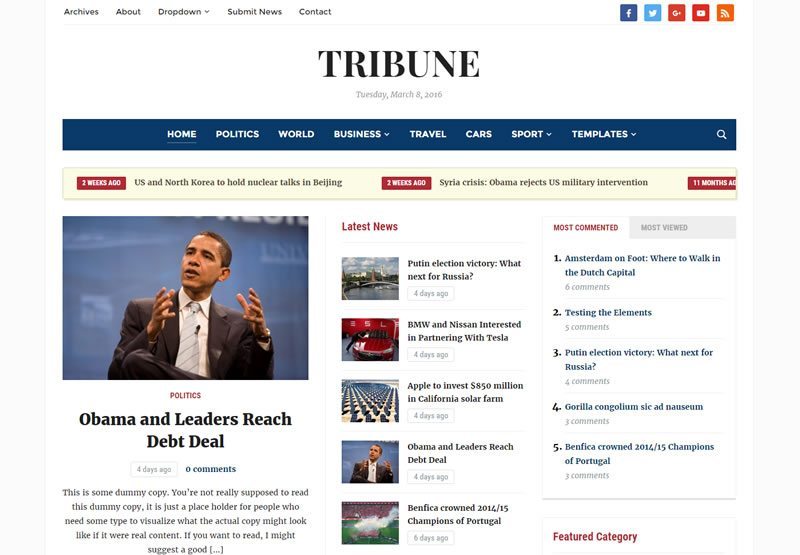A screenshot captures the homepage of an online news publication, The Tribune, prominently showcasing its masthead. The top navigation menu features several links: Archives, About, Submit News, Contact, and social media icons for Facebook, Twitter, Google Plus, and YouTube. An orange square with a sideways Wi-Fi symbol is also visible. The date displayed is Thursday, March 8th, 2016. 

Beneath the navigation bar, categories such as Home, Politics, World, Business, Travel, Cars, Sport, and Templates are listed. Headlines from recent articles appear, including:

- "Two weeks ago: U.S. and North Korea to hold nuclear talks in Beijing"
- "Two weeks ago: Syria crisis: Obama rejects U.S. military intervention"
- "Obama and leaders reach debt deal."

There is also placeholder text that reads, "This is some dummy copy. You're not really supposed to read this dummy copy. It's just a placeholder for people who need some type to visualize what the actual copy might look like if it were real content."

Additional recent news articles are highlighted, such as:

- "Latest news: Putin election victory. What next for Russia?"
- "BMW and Nissan interested in partnering with Tesla."
- "Apple to invest $850 million in California solar farm."
- "Obama and leaders reach debt deal."
- "Benfica crowned 2014/15 champions of Portugal."

Popular topics like "Most Connected," "Most Viewed," and "Amsterdam on foot: where to walk in the Dutch capital" are also featured. Further mentions include "Testing the elements," "Putin election victory. What next for Russia?" and "Guerrilla Congoleum SLC ad nauseam."